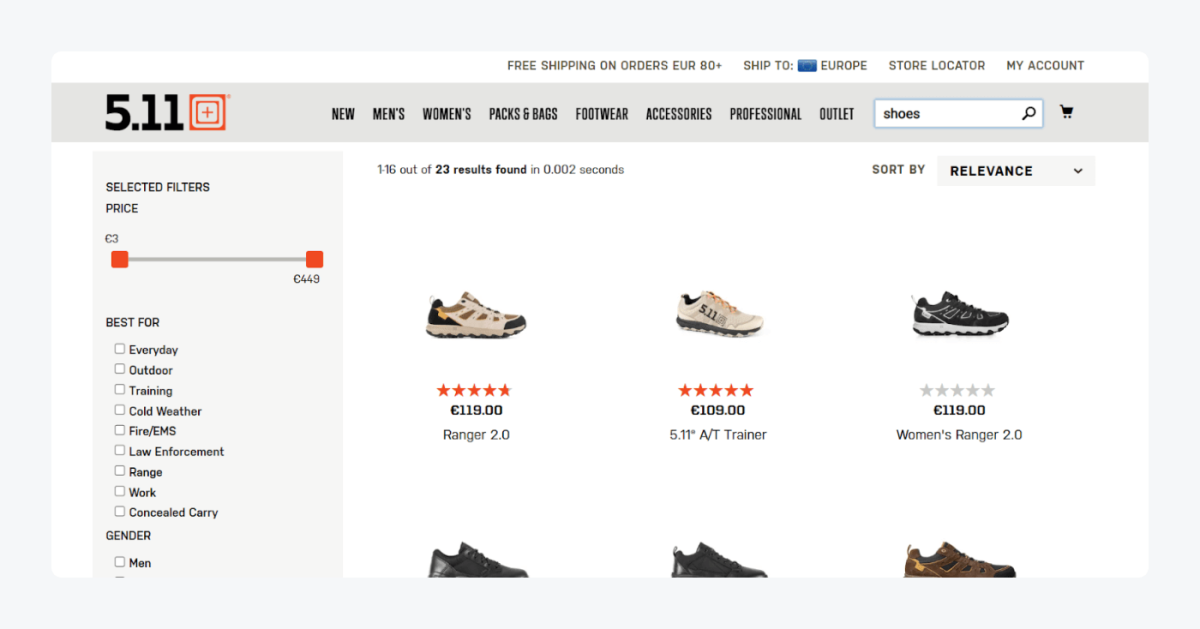Screenshot of an online shoe catalog, possibly from the website 5.11, showcasing various filters and product details. On the left-hand side, there's a navigation panel featuring a slider bar for adjusting price range, currently set from €3 to €449. Underneath, there are additional filters with checkboxes for categories such as "Everyday," "Outdoor," "Training," "Cold Weather," "Fire/EMS," "Law Enforcement," "Range," "Work," and "Concealed Carry." The "Gender" filter is partly visible, with "Men" checked, though other options are truncated and unreadable.

Across the top navigation bar, the site offers free shipping on orders over €80, shipping to Europe, a store locator, and a "My Account" button. Other navigation buttons include "New," "Men's," "Women's," "Packs and Bags," "Footwear," "Accessories," "Professional," and "Outlet."

In the main section of the page, three different shoes are displayed with prices: one at £119, another at £109, and the third also at £119.